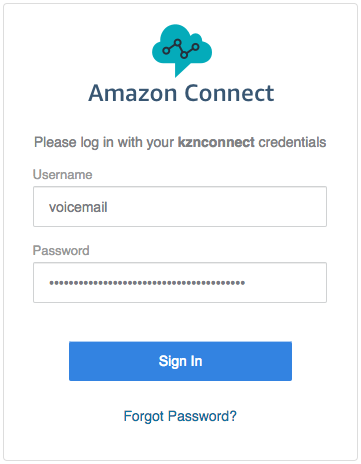The image depicts a gray-bordered rectangle with a white background. At the top, there is a small teal cloud icon connected to three black circles arranged in a zigzag pattern. The first black circle is connected to the teal cloud, with lines angling down and up to the subsequent black circles. 

Below this graphical element, there is a teal arrow pointing downward towards the text "Amazon Connect" in teal. Underneath, in gray text, it says, "Please log in with your kzconnect credentials."

The next element is a text field labeled "Username," consisting of a gray-bordered box with a white interior and the placeholder text "Voicemail" in dark letters on the left side. Below "Username" is another field labeled "Password," followed by a gray box with a series of dark dots, indicating a password entry.

At the bottom of the image, there is a blue rectangular button with the text "Sign In" in white, and below it, in teal text, it says, "Forget Password?" with a question mark at the end.